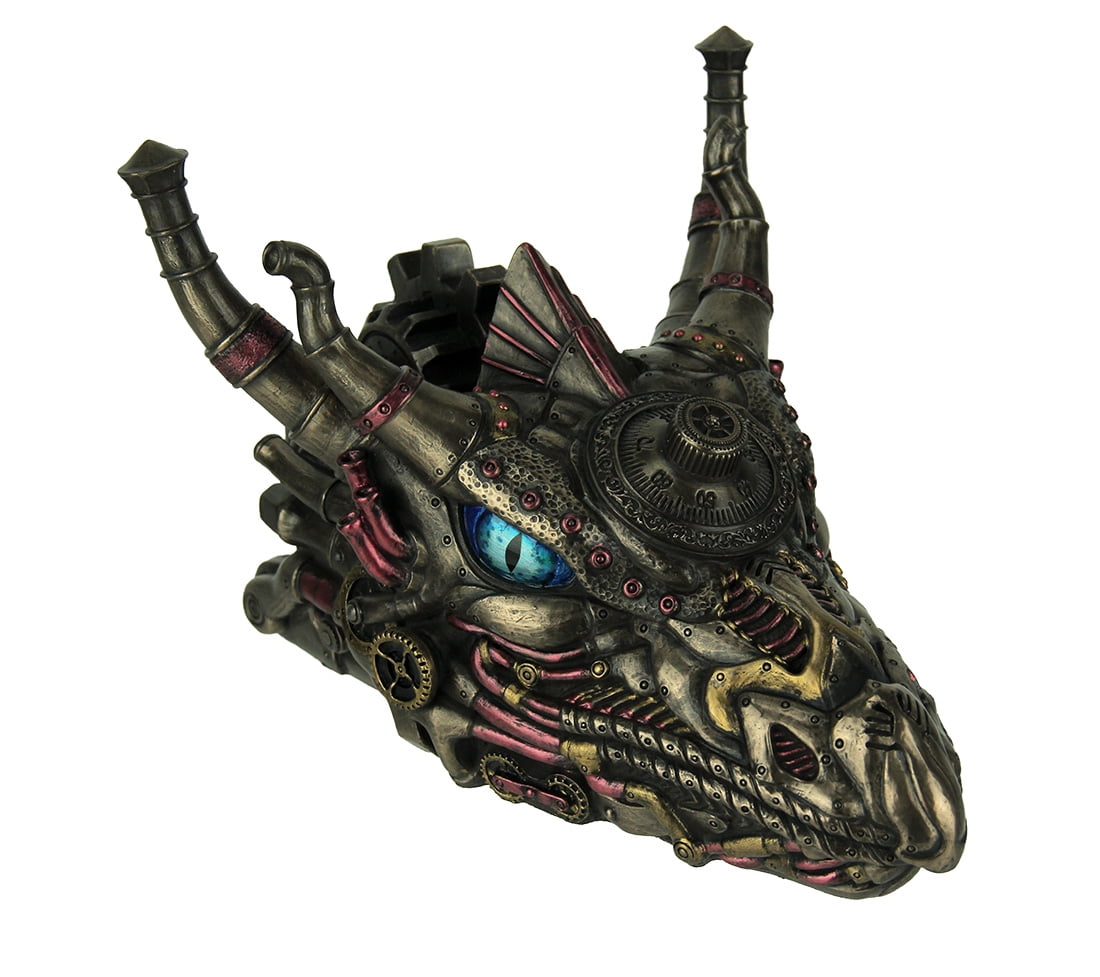The image depicts a highly detailed computer-generated rendering of a dragon head, meticulously constructed from an array of mechanical parts. Predominantly bronze in color, it features striking red metallic accents that complement its formidable appearance. The dragon's eyes are a vivid blue with narrow black slits, reminiscent of a snake's or amphibian's gaze. The dragon's elaborate head features multiple components: its horns are fashioned from interconnected pipes bolted together, giving them a rugged, industrial look; a compass is prominently embedded in the middle of its forehead, adding to the intricate design; the cheeks are adorned with visible gears, while pipes run along the sides of the face, suggesting a complex inner mechanism at work. Additionally, what could be interpreted as ears resemble large chimneys protruding from the head, enhancing its mechanical aesthetic. The presence of a combination lock integrated into the dragon's head further emphasizes the fusion of fantastical and mechanical elements, creating a unique and captivating visual experience.